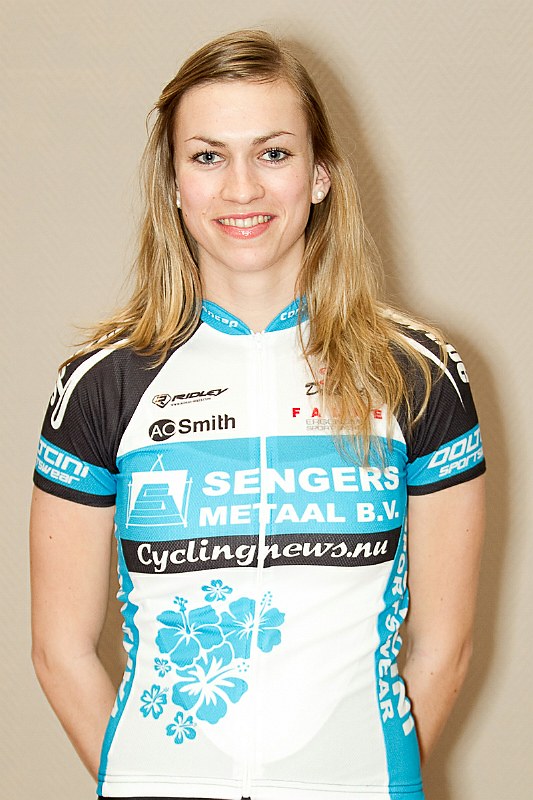A young blonde woman in her early 20s stands confidently in front of a beige background, wearing a cycling suit that highlights her athletic build. Her cycling jersey features a striking combination of colors and text: the shoulders are black, the upper section displays "Senders Metaal B.V" in white font, followed by a thin black bar containing "cyclingnews.nu." The lower section is predominantly white adorned with delicate blue flowers. Her dark eyes and matching eyebrows accentuate her bright smile. She also wears noticeable pearl-like earrings. The image captures her from the waist up, emphasizing the detailed design of her jersey and her composed yet cheerful expression.